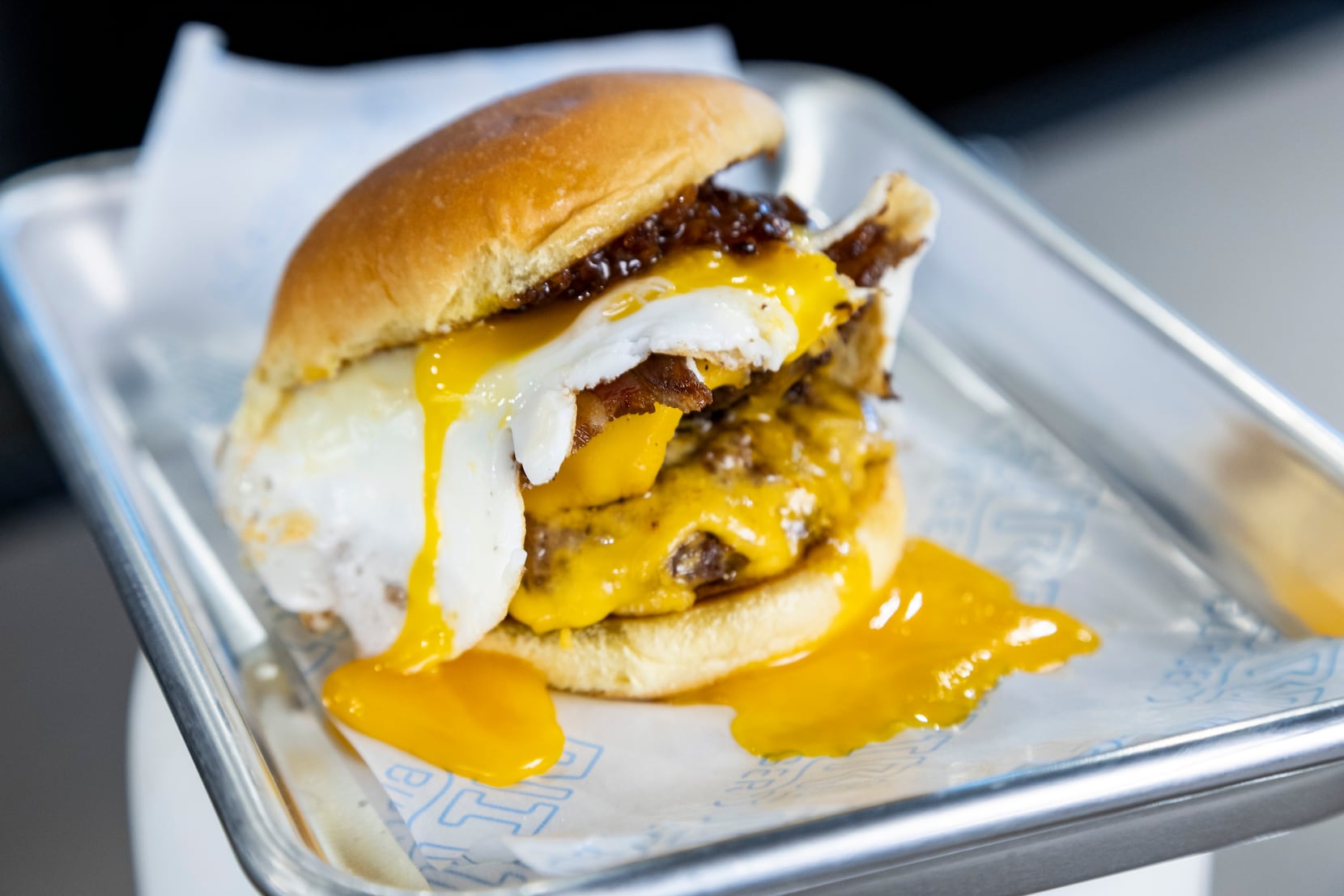In this image, we are looking down at a close-up view of a delectable cheeseburger placed on a silver metal tray. The focus is primarily on the intricately detailed sandwich and its plate, while the background appears blurred. The burger rests on a piece of parchment paper adorned with a light blue, repetitive blocky logo, presumably the brand's name.

The cheeseburger showcases a hearty composition with two well-cooked, juicy hamburger patties, each layered with melted cheddar cheese. Nestled between the patties is crispy bacon, its reddish-brown hue adding a touch of smokiness to the ensemble. Atop the burger sits a perfectly cooked over-easy egg, its yolk luxuriously oozing down the sides of the burger, pooling on the parchment paper both in the front left and bottom right areas of the tray. The sandwich is enclosed with a browned bun on the top and bottom, completing this towering, mouth-watering creation. The rich, marbled sauce drizzling over the egg adds an extra layer of flavor and visual appeal to this indulgent cheeseburger.